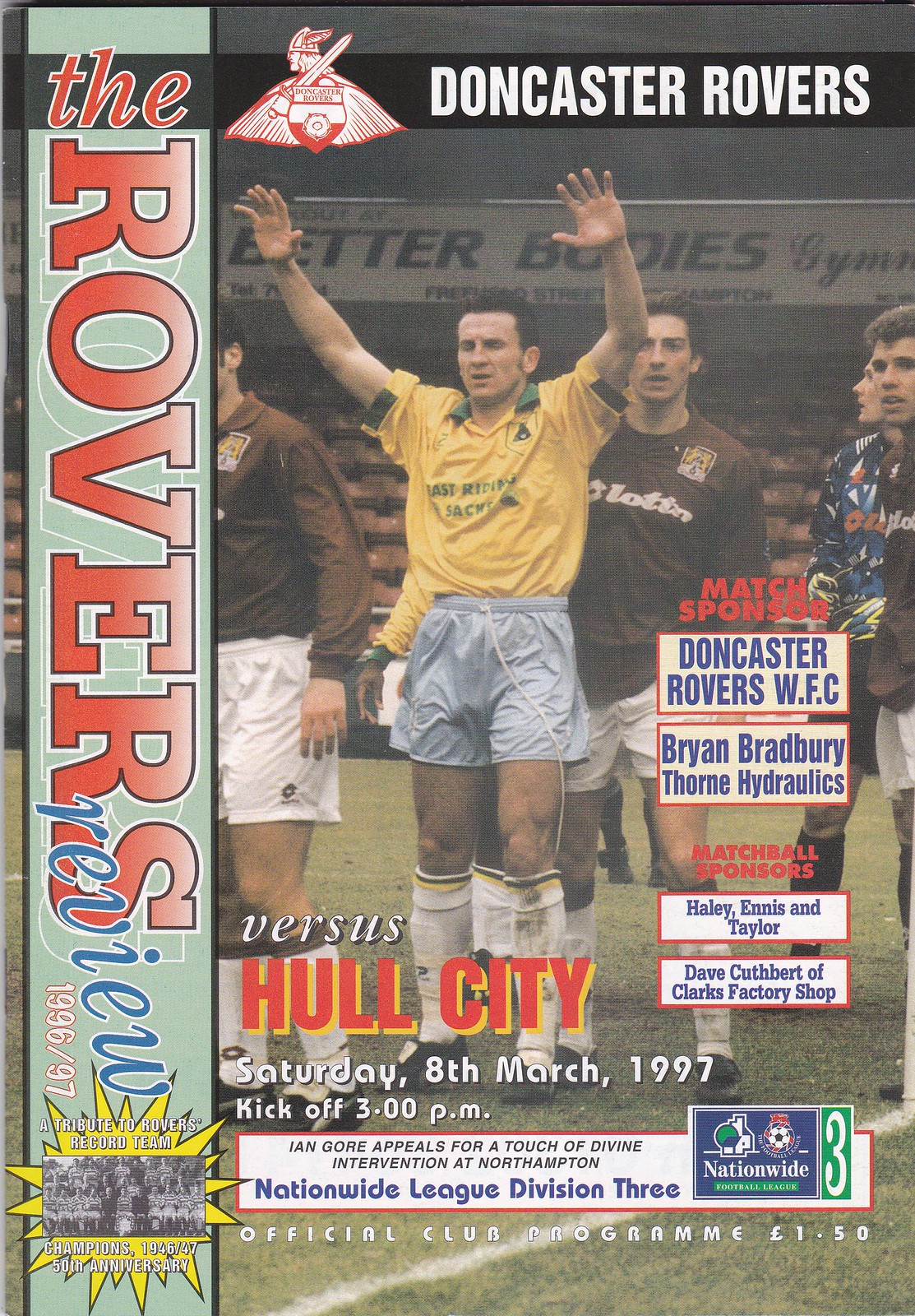This image is a detailed cover of an official Doncaster Rovers Football Club program from the 1996-97 season. Prominently displayed at the top of the program is the title "Doncaster Rovers," accompanied by the team’s mascot logo. Running vertically along the left side of the cover is the phrase "The Rovers Review 1996-97."

At the center of the cover, there's a vivid color photograph of a soccer match, likely an archival image from the past. The players are seen in mid-action on the field with one player, seemingly in a gesture of appeal or celebration, holding his hands up. The players are dressed in distinctly colored uniforms: one team in yellow, green, and white, and the opposing team in brown and white. 

Superposed on or positioned next to the photo, the text lists the match details: "Versus Hull City, Saturday 8th March 1997, kickoff 3pm." The program also notes its various sponsors: "Match Sponsor: Doncaster Rovers WFC, Brian Bradbury, Thorne Hydraulics," and "Match Ball Sponsors: Haley, Ennis, and Taylor; Dave Cuthbert of Clark's Factory Shop." Further down, a notable caption reads, "Ian Gore appeals for a touch of divine intervention at Northampton Nationwide League Division 3," alongside a Nationwide logo. The comprehensive nature of this official club program is emphasized with its listed price of "£1.50."

This richly detailed cover not only emphasizes the fanfare surrounding the match but also situates the event within the broader context of the 1996-97 football season.